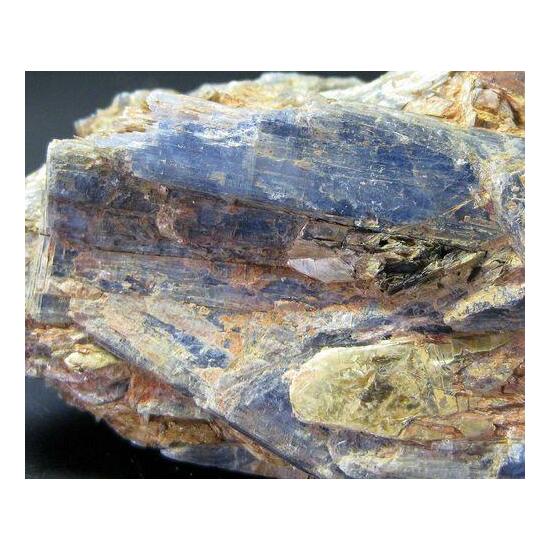The image depicts a close-up view of a single object that could be a slice of wood or a rock, possibly a mineral. Set against a solid black background, the object fills the majority of the square frame and is positioned slightly off-center to the right. Dominated by a palette of various colors including shades of blue, brown, gray, yellow, orange, and hints of gold, the object showcases a mix of flat edges and rougher, textured areas. The upper parts and the middle exhibit flat surfaces, suggesting it has been sliced. The bottom right and lower left regions are more jagged and irregular. The very top of the object features a textured surface reminiscent of small rocks. The overall appearance is speckled and striped, adding to the complexity of its surface. No text is present in the image, maintaining focus entirely on the rich details of the object, which could be part of a geological study, possibly in a museum or archaeology center.